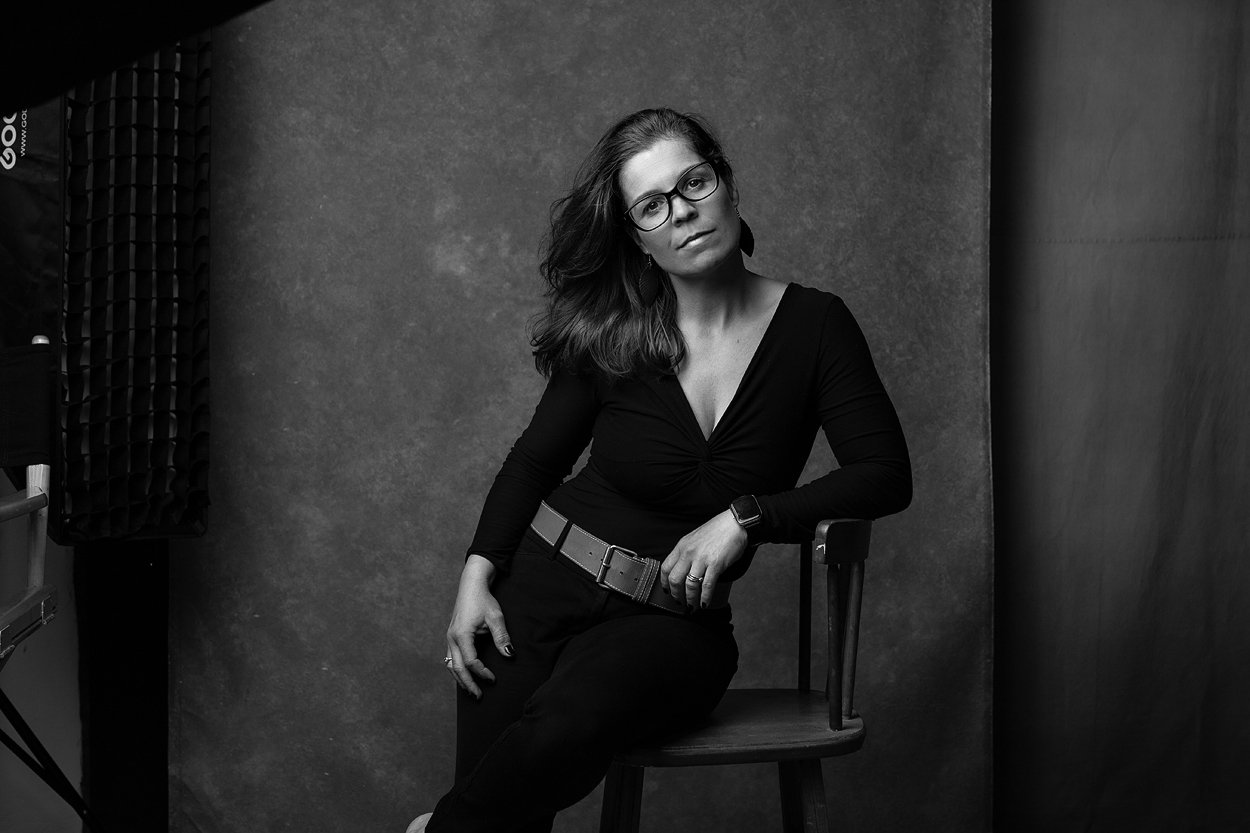In this black and white photograph, a woman is prominently posed in the center. She is somewhat sitting sideways on a wooden chair, with her left elbow resting on the backrest and her hip leaning against the seat. The chair faces to the side while she looks directly at the camera, creating a poised yet relaxed stance. Sporting black-rimmed glasses, her slightly wavy, shoulder-length dark hair is parted to the side.

She is dressed in a V-neck long-sleeved black shirt, accompanied by a thick brown belt that cinches her outfit composed of black pants. Her left wrist features a square-shaped smart device, and she has rings on both of her ring fingers, with nails painted in dark polish. A subtle yet textured backdrop, varying in gradients from light to dark, forms the background of the image. The scene also includes a black director's chair with black fabric and light brown wooden armrests, visible in the bottom left corner, while a net-like plastic square hangs in the top left part of the image, adding a touch of abstract structure to the composition.